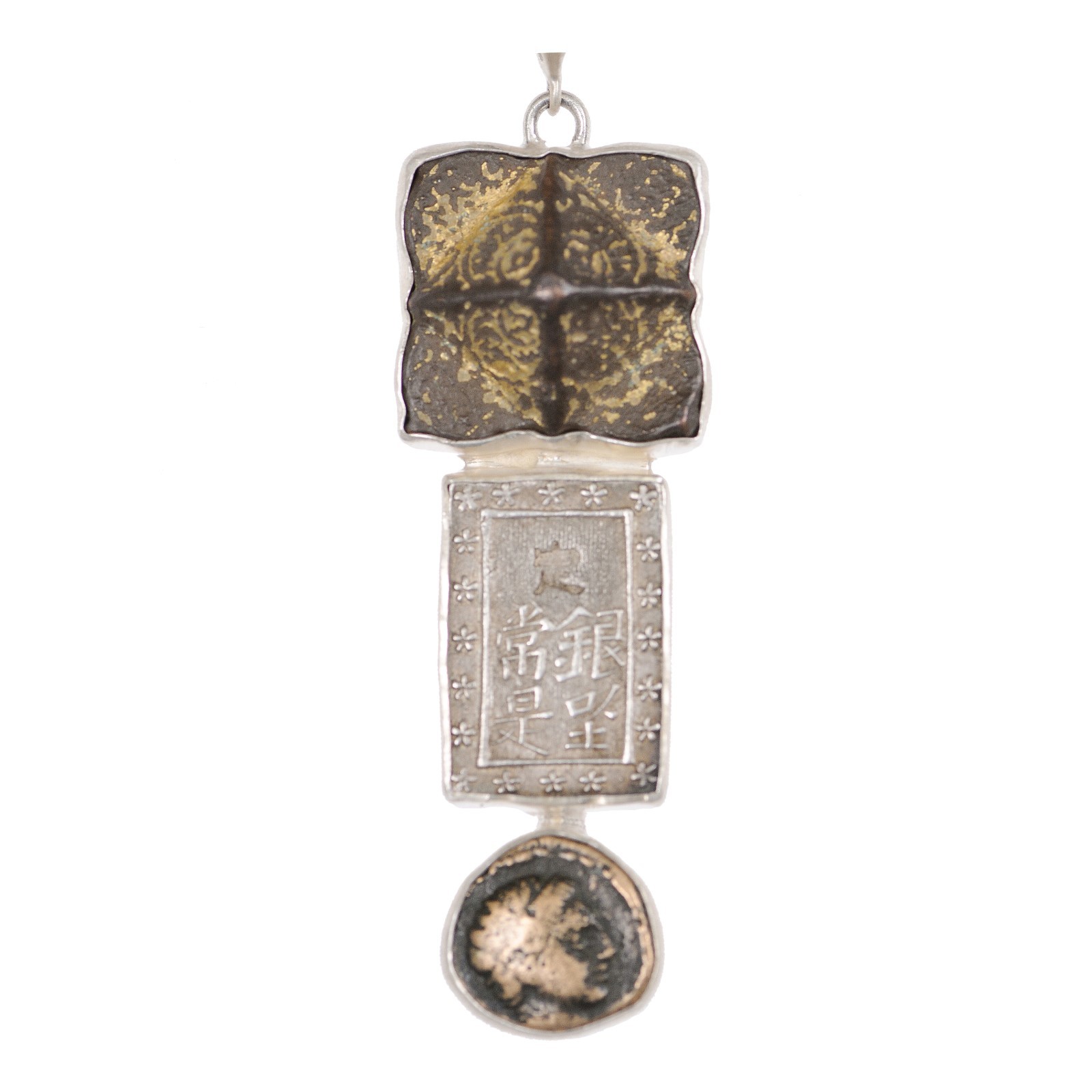The image depicts an antique-style pendant set against a plain white background. At the top of the pendant, a silver loop connects it to a chain. The pendant's uppermost section is a vaguely square-shaped piece of metal, featuring a central cross that divides it into four sections. This squarish piece has a brown and gold inlay with a bronze pyramid-like design cross that stretches vertically and horizontally. Surrounding this cross motif are intricate wavy lines, and the corners exhibit some chipping and aging, adding to its antique charm.

Below the square section, there is a rectangular bracket made of silver metal. This rectangular piece is adorned with Asian characters, possibly Chinese or Japanese, and is bordered with a silver flower design, enhancing its ornate appearance.

The lowest part of the pendant is a round, worn-looking piece of metal. This circular segment appears to be made of bronze, exhibiting both shiny and dull, blackened areas, reflecting its aged nature. The center of this round piece features a rough design that includes a faint imprint of a face. Collectively, these components form a pendant that combines elements of different shapes and intricate designs, unified by a connecting silver metal.